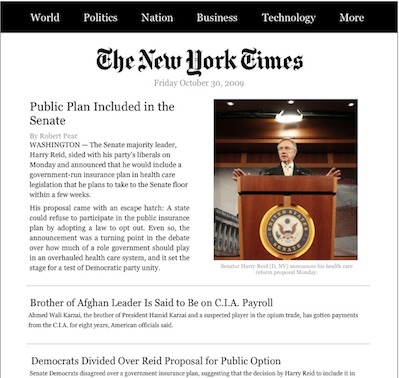A screenshot captured on a smartphone displays the homepage of The New York Times website, dated Friday, October 30th, 2009. The screen features a black banner running across the top with white text that includes categories such as World, Politics, Nation, Business, and Technology. Beneath the banner, the iconic New York Times name is presented in a large, old-style black font, with the date written in a more regular grey font underneath.

Dominating the left side of the screen, a headline in black font reads, "Public Plan Included in the Senate," followed by the author's name and two brief paragraphs summarizing the article. Adjacent to the text, on the right side, is a photograph featuring a man with grey hair standing behind a podium. The podium is adorned with the official seal of the United States Senate, depicting an eagle with outstretched wings. Below this image, titles of two additional articles are listed, providing a glimpse of the other news featured on the site.